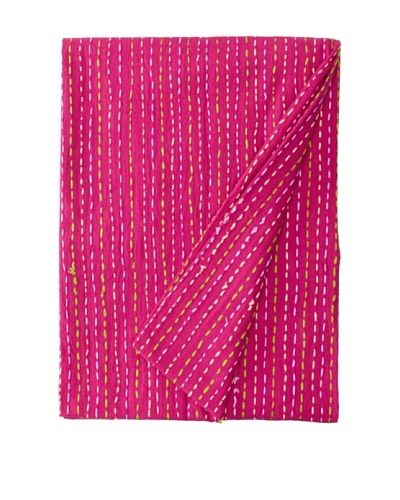A neatly folded piece of fabric occupies the entire image, set against a pure white background. The fabric is predominantly a dark pink or fuchsia color, but some may describe it as a light red. It features a pattern of vertical lines that alternate between different colors, including white, yellow, and potentially shades of blue, green, and purple. These lines run from top to bottom and are unevenly spaced, adding an element of playful irregularity. One corner of the fabric is folded back, revealing an identical underside with the same colorful vertical stitching. The lines appear to differ in spacing and color, giving the fabric a dynamic, non-uniform look. The background is entirely white, potentially suggesting it was either extremely bright or digitally removed. The exact use or size of the fabric remains uncertain—it could be anything from a shower curtain to a tablecloth or even a dishcloth.